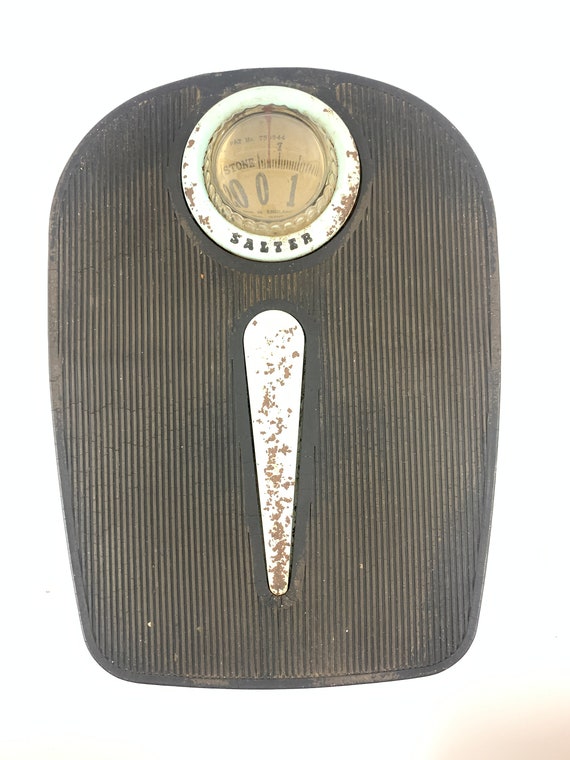The image depicts an old-fashioned, well-worn body weighing scale prominently placed against a solid white background. The scale features a rectangular shape with a rounded top, where a circular dial displays the numbers. This dial, outlined by a silver band, appears aged and worn, with some faint, indiscernible text. The brand name "Salter" is clearly visible below the circular area. The scale surface is black with ridges running horizontally across it to provide traction and grip. In the center of the scale, a vertical white stripe, resembling an exclamation mark without the dot, serves as a guide for foot placement. The red indicator line, which shows the measured weight, is poised at zero in the circular dial, ready to move when someone steps on the scale.